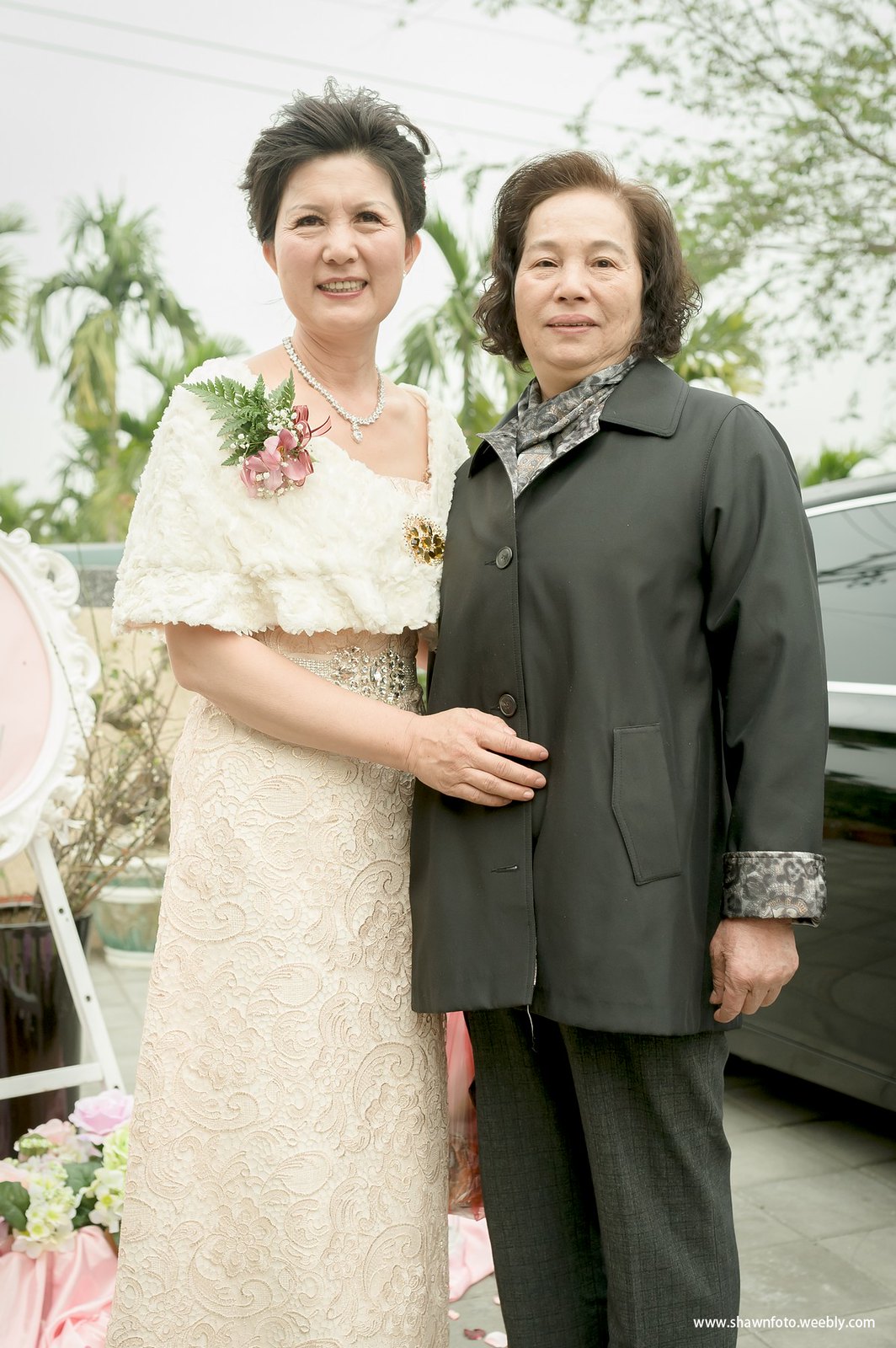In this detailed outdoor photograph, two middle-aged women are posing and smiling at the camera. The scene is set against a backdrop of green trees and a hazy sky, with power lines visible overhead. The woman on the left is dressed in a very ornate, white fluffy gown with a floral design, reminiscent of a wedding dress. She accessorizes with a pearl necklace, a corsage featuring pink flowers and green ferns on her right shoulder, and a silver brooch or belt at her waist. Next to her stands the woman on the right, who has short brown, medium-length hair and wears a dark jacket with patterned, rolled-up sleeves paired with dark plaid slacks. In the background, a black sedan is parked on what appears to be a paved driveway, adding to the casual yet celebratory ambiance. A white and pink easel or picture frame stands partially visible behind them, along with a cluster of flowers on the ground near the woman in the gown. The women, both smiling and adorned with corsages, suggest a special event or celebration. At the bottom right corner of the image, the watermark "www.seanphoto.weebly.com" is faintly visible.